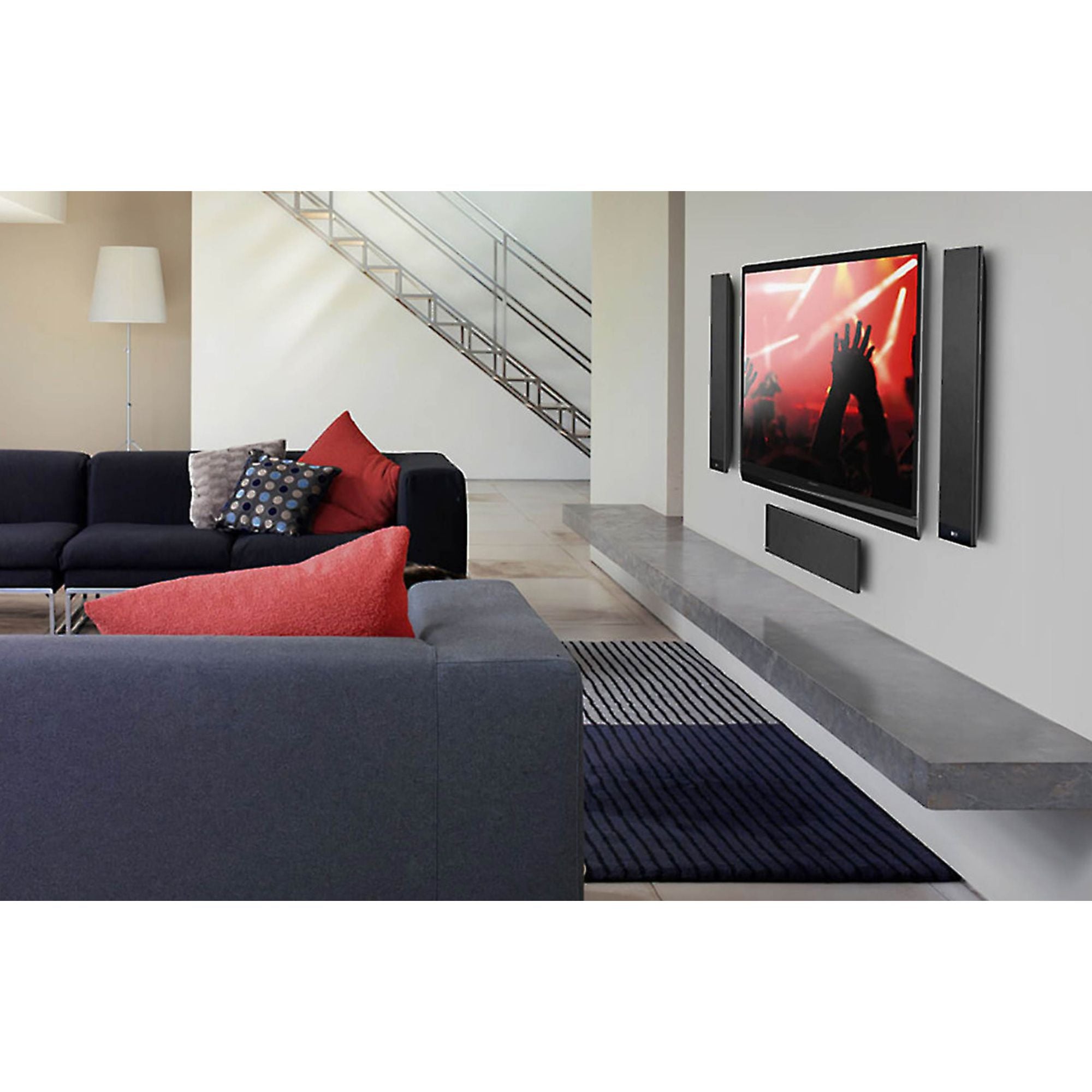This image depicts a modern living room characterized by a light gray wall on the right, dominated by a large flat screen TV flanked by black rectangular speakers on either side and another speaker below it. Directly beneath the TV, there is a wide, floating gray marble or granite countertop extending across most of the wall. The floor below features a bi-color rug, primarily white on the top half and blue on the bottom half, adorned with horizontal lines.

On the left side of the room, two sofas face each other: the one closest to the viewer is dark gray, while the farthest sofa is black. Both sofas are adorned with red throw pillows, and the black sofa also has a gray pillow and a black one with multi-colored circles. Towards the center top of the image, a sleek metal staircase ascends, contrasting with the white wall behind it. In the far top left corner, a white floor lamp with a matching lampshade adds to the room's modern aesthetic.